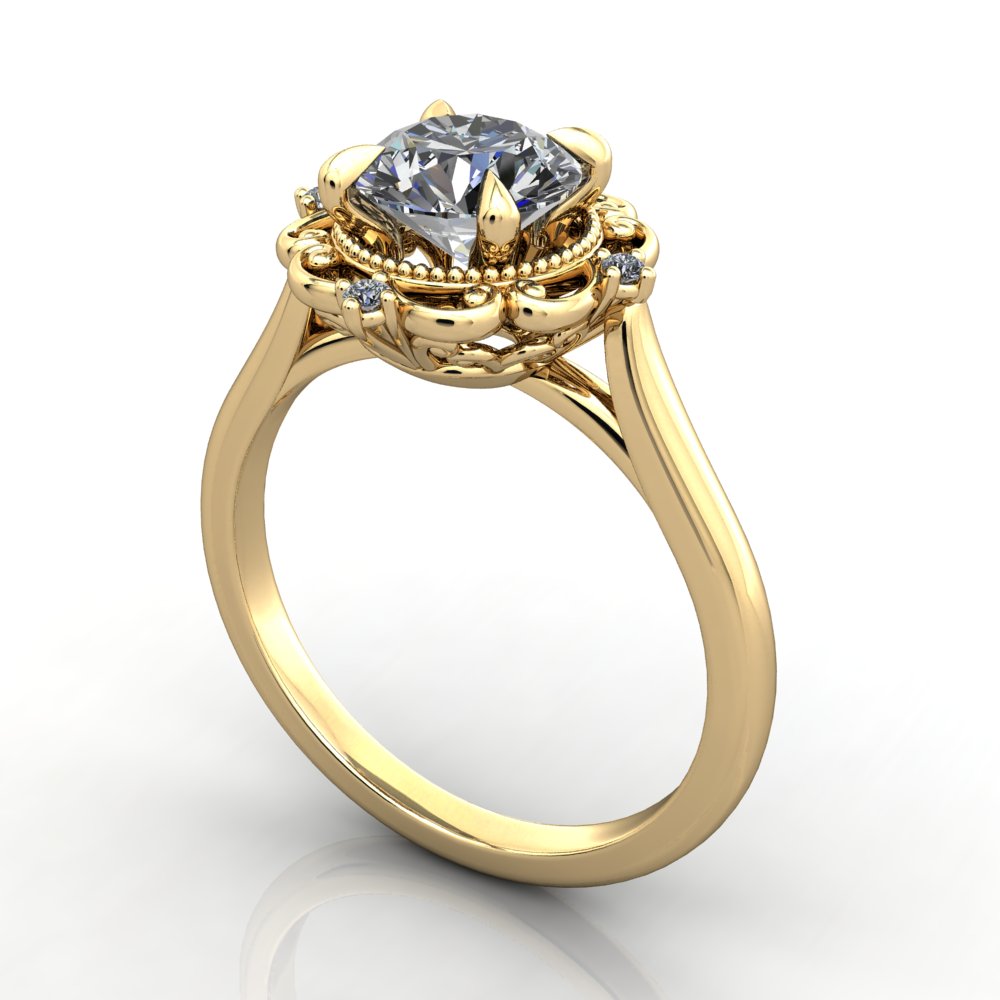The image showcases an intricately designed gold ring set against a glossy, reflective white background. The prominently featured diamond at the center is held securely by four gold prongs, creating an open space around its bottom edges. The diamond has a whitish to grayish-blue hue, adding to its brilliant allure. Surrounding the central diamond, smaller diamonds are similarly held by four prongs. Adding to the ring's elaborate design are tiny golden beads and ornate, vinish patterns, along with a heart shape nestled near the diamond. Beneath these elements is a delicate flower design, further enhancing the ring's exquisite craftsmanship. Subtle gray shadows and strategic lighting draw attention to the ring’s detailed artistry, which appears almost too perfect, suggesting the image may be a computer-generated render.